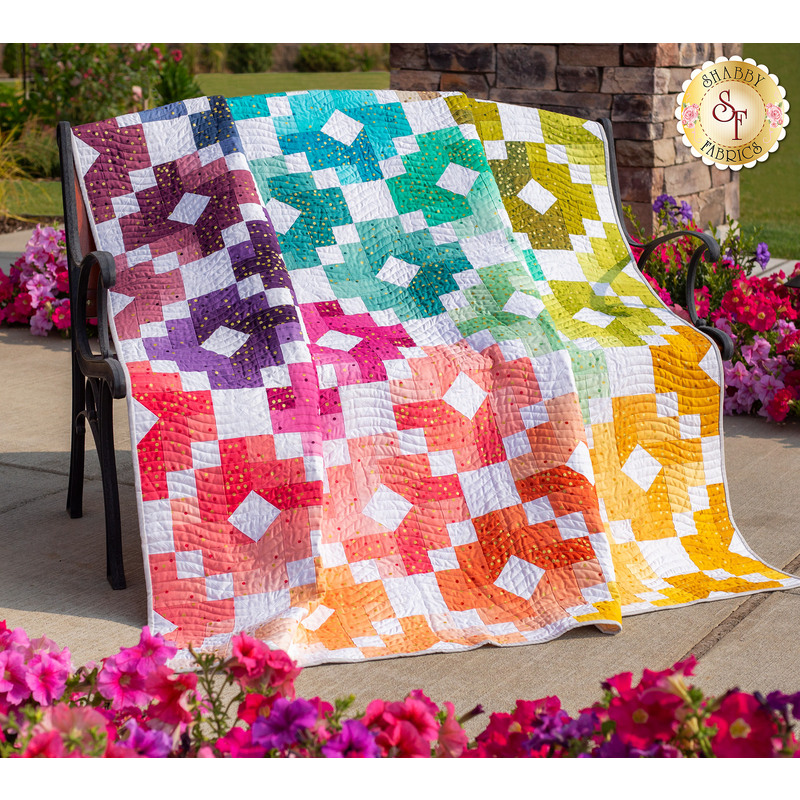This professionally taken photo captures a beautifully maintained garden scene, centered on a stylish wrought iron black bench. The bench is draped with a multicolored patchwork quilt that obscures its upholstery. The quilt has a white background with vibrant squares featuring shades of pink, purple, violet, red, orange, yellow, green, blue, and peach, creating a rainbow effect. The geometric patterns include white triangles and colorful squares, divided into prominent sections: the left showcasing purples and reds, the middle with greens and oranges, and the right dominated by bright greens and yellows.

The bench rests on a cement floor made of large square tiles. Surrounding the bench is a lush garden adorned with pink and purple flowers both in the foreground and background. Behind the bench, there's a stone wall displaying a mix of black, white, gray, and brown shades. A brick column is visible on the right side of the image, adding to the garden's structured aesthetic. Green grass occupies the upper part of the picture, completing the serene outdoor setting.

In the upper right corner of the image, a gold emblem with the inscription "shabby fabrics SF" signifies the professional and curated nature of the setup. The overall composition captures the essence of a thoughtfully designed and well-maintained garden area, possibly part of a renowned estate.